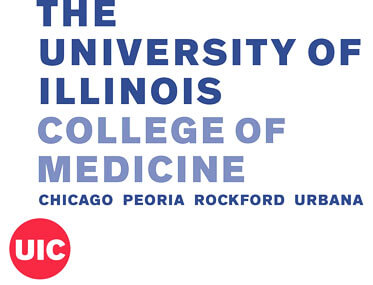The image appears to be a textual graphic from a webpage, possibly serving as a header or part of a larger layout. It features several lines of text, meticulously arranged and color-coded. Here's a detailed breakdown:

1. **Text Arrangement and Color:**
   - The top three lines are in all caps, dark to medium blue, with left-justified alignment:
     - **First Line:** "THE"
     - **Second Line:** "UNIVERSITY OF"
     - **Third Line:** "ILLINOIS"
   - The next two lines are a lighter blue with the same left-justified alignment:
     - **Fourth Line:** "COLLEGE OF"
     - **Fifth Line:** "MEDICINE"
   
2. **Additional Information:**
   - Beneath these primary lines, there is a list of locations in the same font but with slightly wider kerning:
     - "CHICAGO, PEORIA, ROCKFORD, URBANA"

3. **Logo:**
   - At the bottom of the text, there is a red circular logo with "UIC" in all caps across its center.

4. **Background:**
   - The entire composition is set against a plain white background.

The overall aesthetic suggests it could be part of a web page header, a section underneath a menu, or an element within a pop-up ad, possibly accompanied by a photo or additional text elsewhere on the page.